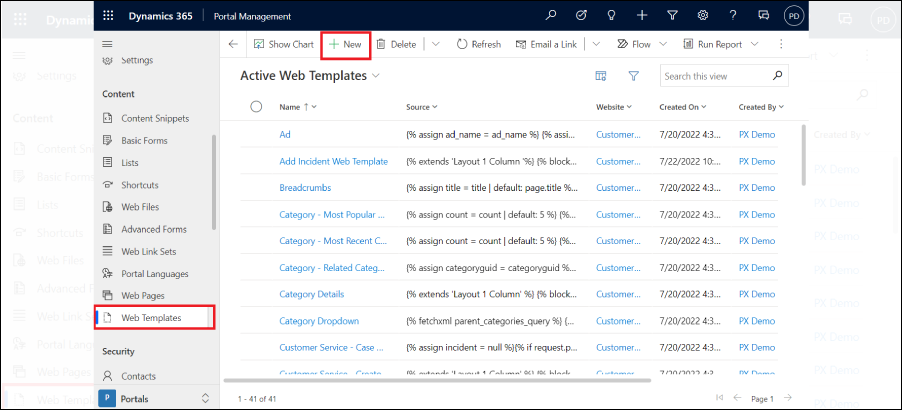The image depicts a webpage interface dedicated to managing web templates within a "Dynamics Portal Management" system. At the very top, the interface title reads "Dynamics Portal Management," establishing the context of the page. Beneath the title lies a navigation menu featuring various options including "Content Snippets," "Basic Forms," "Lists," "Shortcuts," "Web Files," "Advanced Forms," "Web Link Sets," "Portal Language," and "Web Pages." The menu item "Web Templates" is highlighted with a red box, indicating it is currently selected.

On the right-hand side of the interface, within a section labeled "Active Web Templates," a comprehensive list of web templates is displayed. This list includes columns for template names, designations, creation dates, and the individuals who created each template. One specific entry shows the template name "Add" followed by "Design Add Name." The templates in the list all have creation dates such as "7-20-2022," and these dates appear to be consistent across multiple entries.

Above the template list, there are several action buttons: "Show Chart," "New," "Delete," "Refresh," "Email A Link," "Flow," and "Run Report." The "New" button is highlighted with a red square, indicating that the user has selected the option to create a new template. Additionally, at the top-right corner of the page, there is a search box, allowing users to easily search for specific templates.

Overall, this screenshot provides a detailed look at the administrative interface used for managing web templates within the Dynamics Portal Management system.